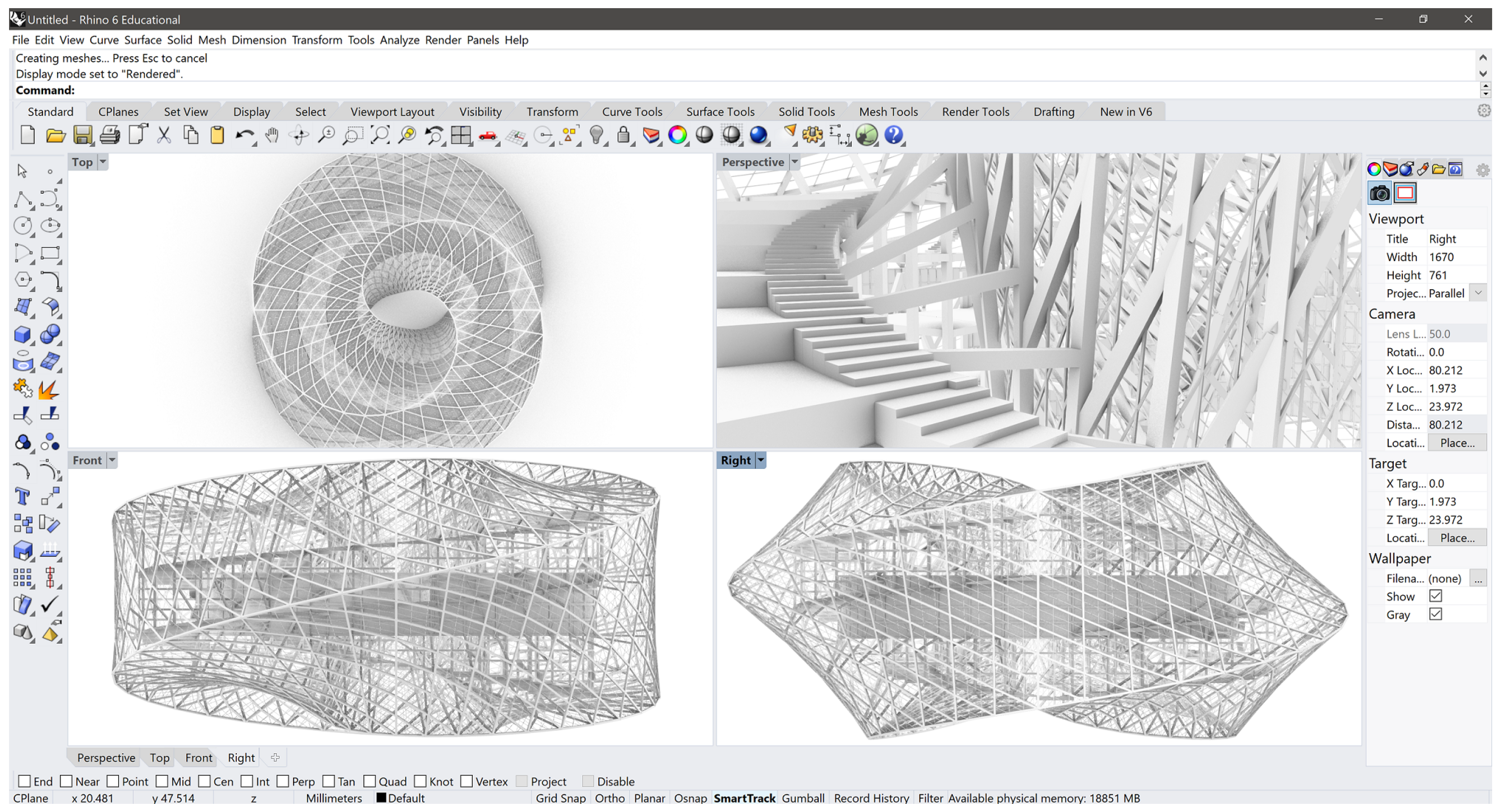This image is a detailed screenshot of a computer screen showcasing a 3D design project within the "Untitled-Rhino 6 Educational" application on a Windows operating system. At the top, the classic Windows interface displays the file name and the standard control buttons (Minimize, Maximize, Close). Directly below, the software menu bar includes options like File, Edit, View, Curve, Surface, Solid, Mesh, Dimension, Transform, Tools, Analyze, Render, Panels, and Help. The workspace is divided into four quadrants, each providing a different perspective of the design: Top, Perspective, Front, and Right. These views collectively depict a complex structure, mainly a white spiral staircase surrounded by numerous beams and support bars. Surrounding the central work area are various toolbars containing a multitude of icons and shortcuts. The left side features two columns of tool icons, while the right side provides detailed information about the project, including camera coordinates and viewport dimensions. At the bottom, a series of clickable checkboxes labeled End, Near, Point, Mid, etc., offer additional functionalities. The overall interface is densely packed with features, reflecting the application's advanced capabilities for professional 3D design and engineering work.